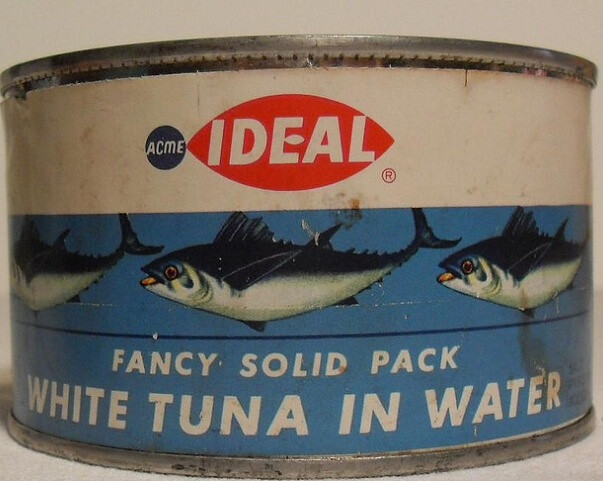This image depicts a vintage tin of tuna, characterized by its aged appearance and outdated design elements. The can is made of silver metal, featuring prominent rims at the top and bottom, and exhibits signs of wear and age. The label is notably worn and not in the contemporary style of modern canned tuna labels, suggesting it is from an older era.

The label itself includes several distinctive features. At the top, a white band encircles the entire can. Within this band, a black circle is prominently displayed, containing the word "Acme" in white lettering. Adjacent to this, there is a red, fish-shaped emblem with the word "Ideal" in white, accompanied by a red "R" at the bottom, encircled.

On the main part of the label, a vibrant blue background showcases an illustration of three tuna fish swimming. Below this illustration, in bold white uppercase letters, the text reads "Fancy Solid Pack White Tuna in Water," specifying the product type. The background around the can is plain, without any additional objects or scenery, keeping the focus solely on the vintage tin of tuna.